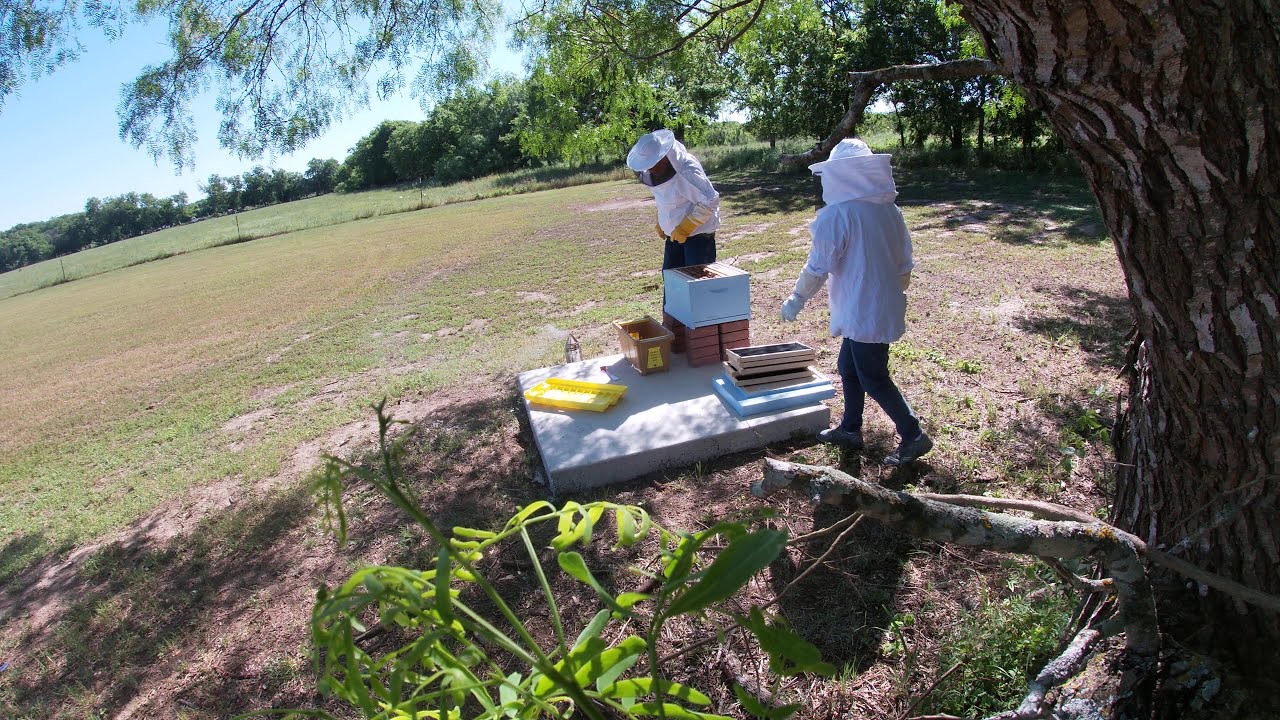The photo depicts a sparse, open space outdoors that could be a park or a backyard. The grass is light green and patchy, with areas of brown dirt showing through. In the foreground, at the center, a green plant stands out, while to the right, there is a robust tree with thick roots visible above the ground. Two people, dressed in partial beekeeper uniforms consisting of white tops, white gloves, and brimmed hats with face coverings, are engaged in beekeeping activities. 

The scene's focal point is a small, raised concrete platform in the center, home to several beehive boxes. One of the beekeepers, possibly a woman, is walking towards the platform and wearing gray pants and a large white jacket. Several rectangular beekeeping tools, including a light blue box with a brown, ridged container resembling a basket on top, lie near her. The other beekeeper, likely a man, is bent over, working with another box, seemingly organizing or extracting something. There are additional beehive components, including extra flat trays and a yellow plastic lid, scattered nearby on the platform.

In the background, further under an overhang of trees, there is more lush, green grass, contrasting with the patchier foreground. A fence post and thicker foliage with green leaves are visible even further back, creating a natural boundary for the open space. The scene suggests an active beekeeping operation during what appears to be midday under a bright sky.